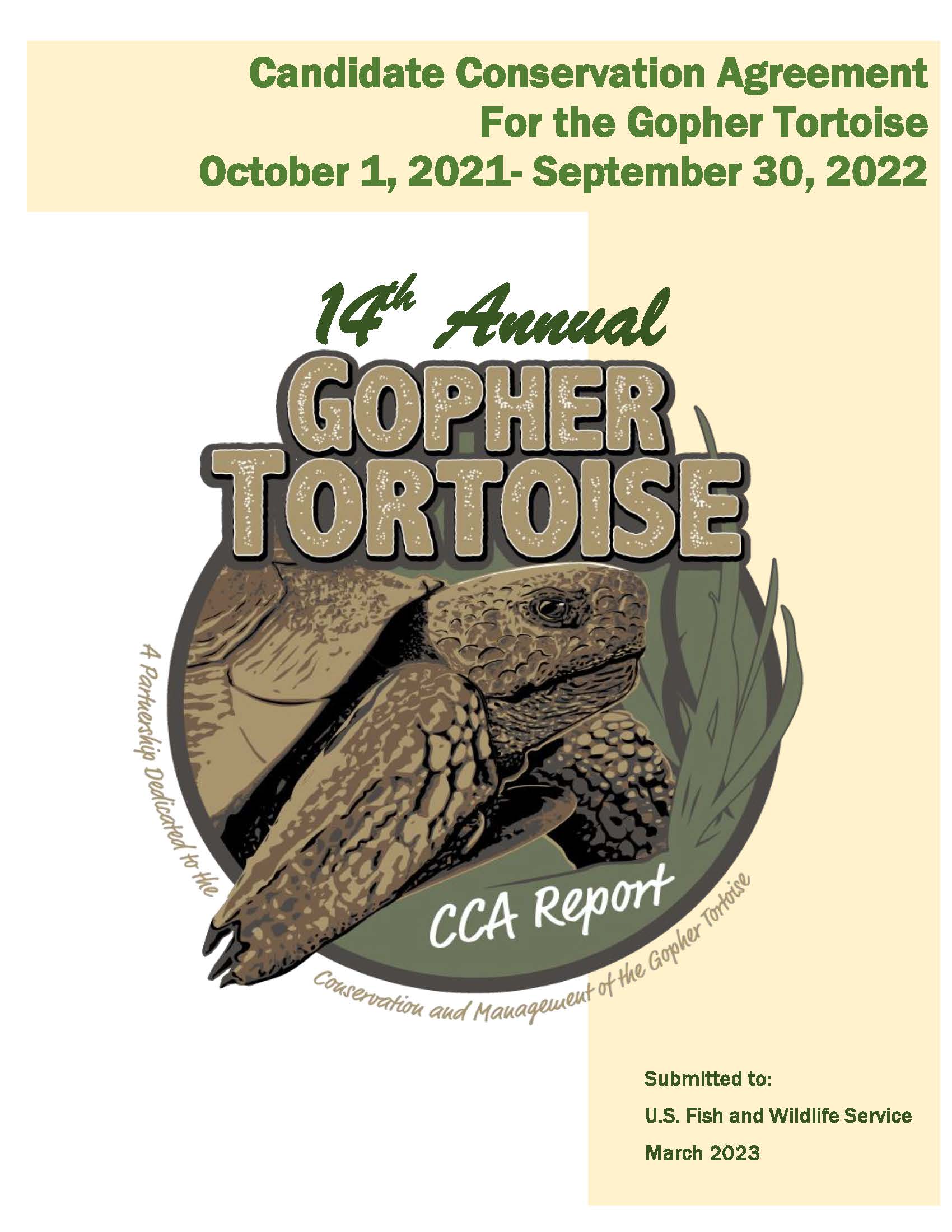The image features a sign with a dual-colored background: white on the left and a light peach color extending along the top and right side. At the top, in olive green font, it states, "Candidate Conservation Agreement for the Gopher Tortoise" with the dates "October 1, 2021 – September 30, 2022" directly beneath. Central to the design is a dark olive green circle containing a drawn image of a gopher tortoise, which is facing to the right. The tortoise, rendered in shades of tan and green, has one flipper extended beyond the circle’s boundary. The circle also features silhouettes resembling underwater grass on its right side. Above the tortoise, in olive green font, it reads "14th Annual," and below in large, olive-tan block letters, "Gopher Tortoise." At the base of the circle, in white font, it says "CCA Report," accompanied by the text "A partnership dedicated to the conservation and management of the Gopher Tortoise" in tan lettering. Finally, at the bottom right corner in small olive green font, it notes, "Submitted to U.S. Fish and Wildlife Service March 2023."